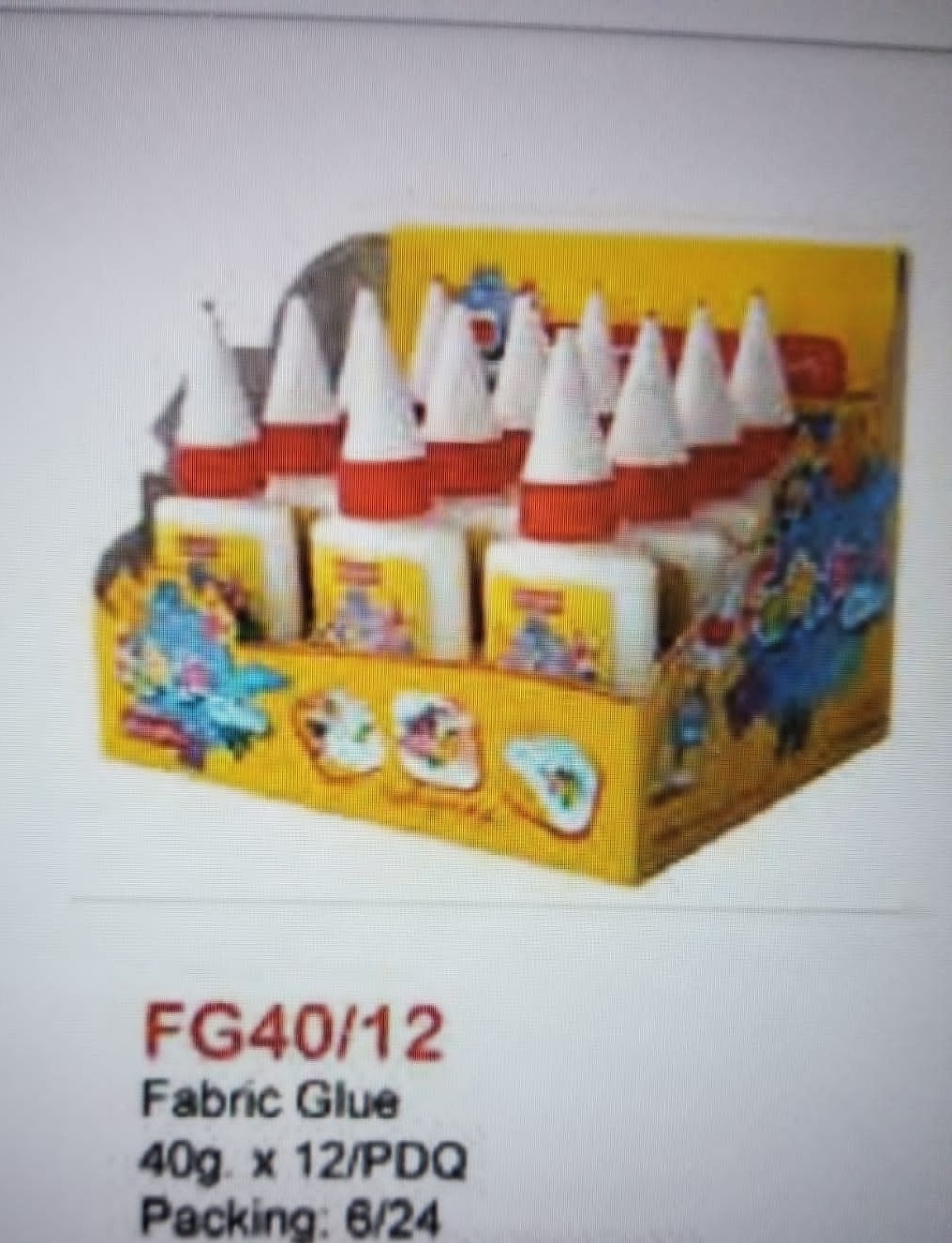This image appears to be a slightly blurred photograph of a catalog or website page showcasing a product. At the top of the picture, there's a line or possible crease, slightly tilted down towards the right, suggesting it's the top of a page being turned. The rest of the image background is predominantly white with some shadowing, reinforcing the impression of a page crease.

The focal point is a set of 12 bottles of glue. Each bottle features a yellow label with colorful accents, and the bottle itself is white. The glue bottles have cone-shaped tips, designed for precision application, which are white in color. A red screw cap secures the tip to the bottle.

The glue bottles are housed in a carton with a design that includes various colors like blue, pink, and yellow, although the exact patterns are unclear due to the image quality.

Below the image of the glue carton, there is product information text: "FG40-12. Fabric glue, 40 grams x 12 / PDQ packing 6-24." This indicates that each bottle contains 40 grams of fabric glue, and the packaging method is "PDQ packing 6-24."